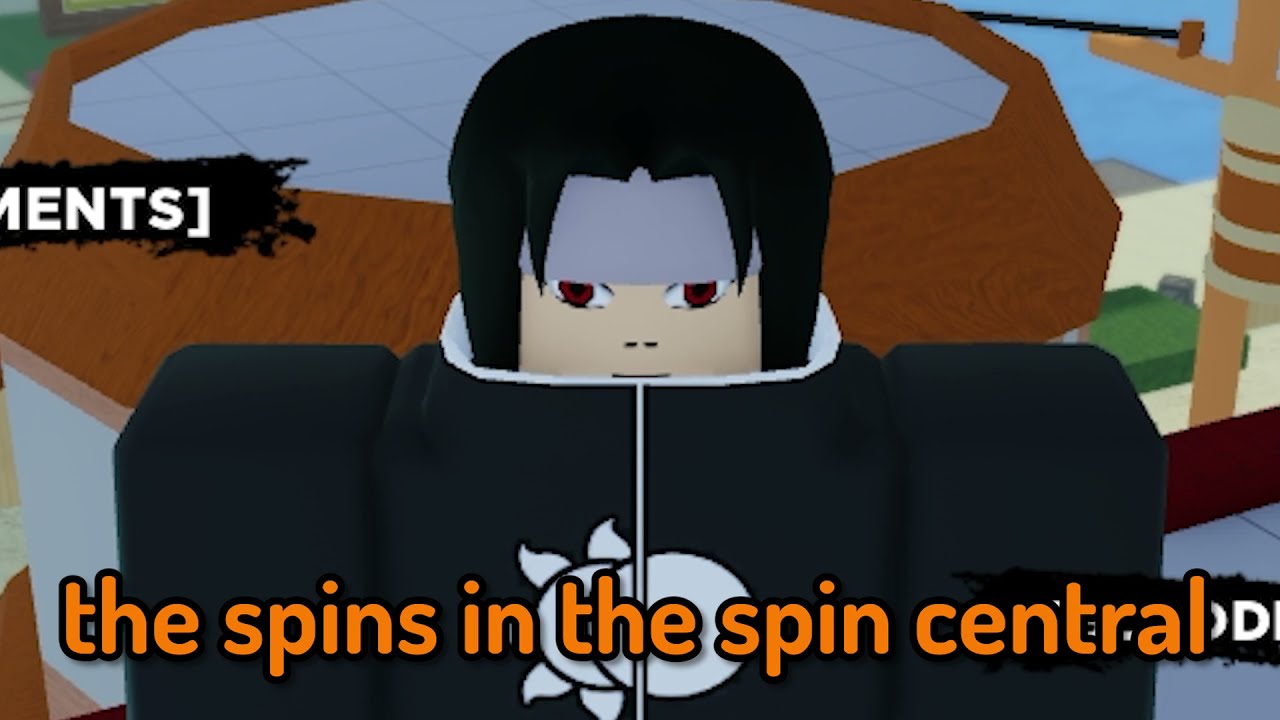The image appears to be a screenshot from a cartoon or video game featuring an anime-style, cartoony portrait of an Asian man or boy with long dark hair. He is wearing a gray bandana that covers his eyebrows, revealing his striking red or orange eyes. His skin tone is medium, and he is dressed in an oversized, dark gray football or robotic uniform with exaggerated, blocky shoulders, shown from head to about the armpits. The uniform features a white double sun logo on the front. The character's head is barely peeking out over the high collar of the uniform, with only his mouth and eyes visible.

The background is somewhat ambiguous, depicting what seems to be the top of a building with a glass or transparent roof, possibly resembling a greenhouse, set against a body of water. Elements in the background include a pole with brown stripes, perhaps resembling a telephone pole. Text in black and white can be seen in the upper left corner, displaying "MENTS" with closing quotes or parentheses.

On the bottom of the image, there is prominent orange text reading "The Spins in the Spin Central," stretching almost from the left edge to the right edge. The overall scene gives a sense of a futuristic or game-like universe.